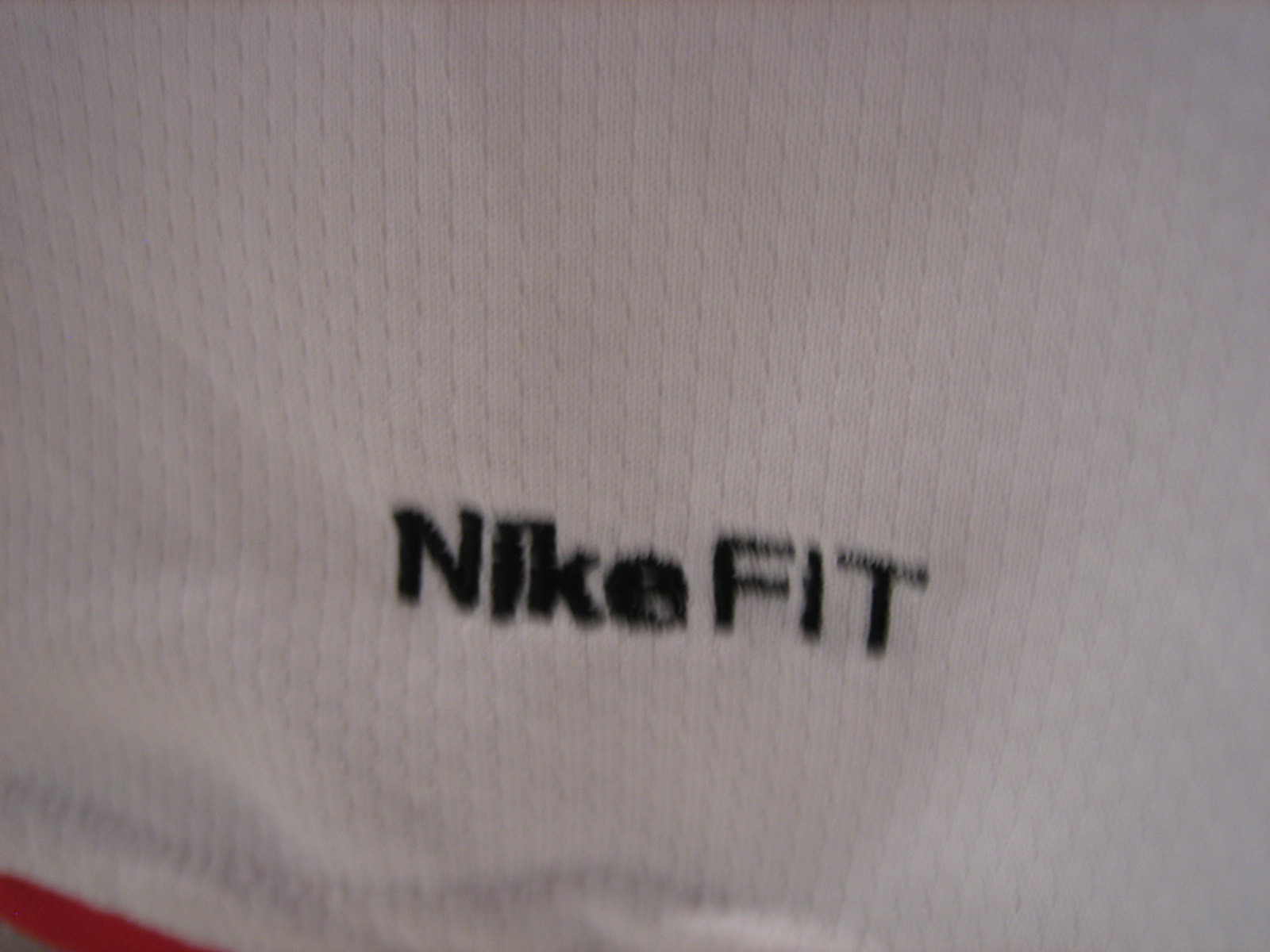This indoor close-up photograph showcases a piece of white, breathable knit fabric with a detailed texture reminiscent of a tech material, possibly from clothing like a top, leggings, underwear, or even socks. The fabric spans the entire image, appearing from the left to the right and from the top to the bottom, except for a portion in the lower left corner where a red stripe runs diagonally. The fabric features a hexagonal pattern stitched throughout. Centered below the midpoint of the frame, the blurry but visible black embroidery reads "NIKE FIT" with 'NIKE' in a combination of thick and thin letters and 'FIT' in thin capital letters. There are no other logos or words visible, suggesting the intent to highlight the authenticity of this Nike product. The image quality is poor, dimly lit, and slightly out of focus, yet the NIKE FIT embroidery remains distinguishable against the textured backdrop.